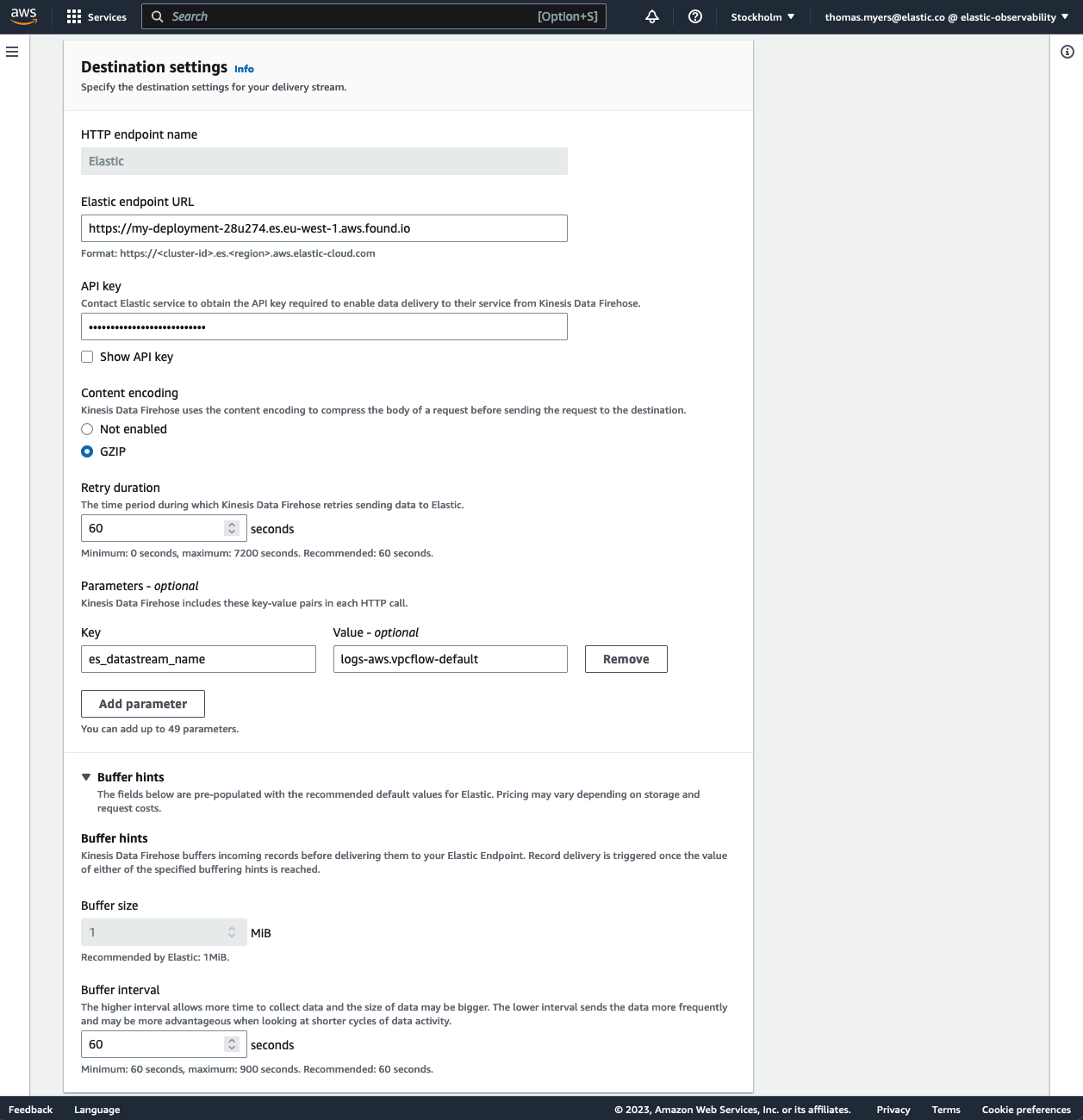Screenshot of a form displaying detailed configuration settings for a delivery stream endpoint on an AWS interface. At the top, the form is titled "Destination Settings" and prompts users to specify settings for their delivery stream HTTP endpoint. Key fields include:

1. **Endpoint Name**: "elastic"
2. **Endpoint URL**: Shows a URL (specific URL not visible in the screenshot).
3. **API Key**: Secured with dot symbols, concealing the text entered.
4. **Content Encoding**: The option "GZIP" is selected.
5. **Retry Duration**: Set to 60 seconds.
6. **Parameters (Optional)**:
    - **Key**: "yes_data_stream_name"
    - **Value**: Displays as a link (specific link not visible in the screenshot).
7. **Buffer Hints**:
    - **Buffer Size**: 1 MIB
    - **Buffer Interval**: 60 seconds

The AWS logo is visible at the top left corner.